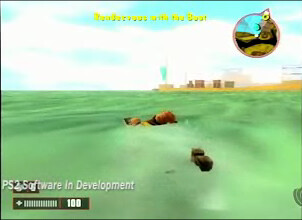This image is a low-resolution, pixelated, and blurry graphical artwork in a square format. At the bottom left, "PS2 software in development" is written in white text. The top middle of the image features yellow text, which is also difficult to discern due to the blurriness. The background showcases a light blue and white sky, with a green-hued body of water below. In the middle of the water, there appears to be an indistinct object or structure, but the poor image quality makes it challenging to determine what it is.